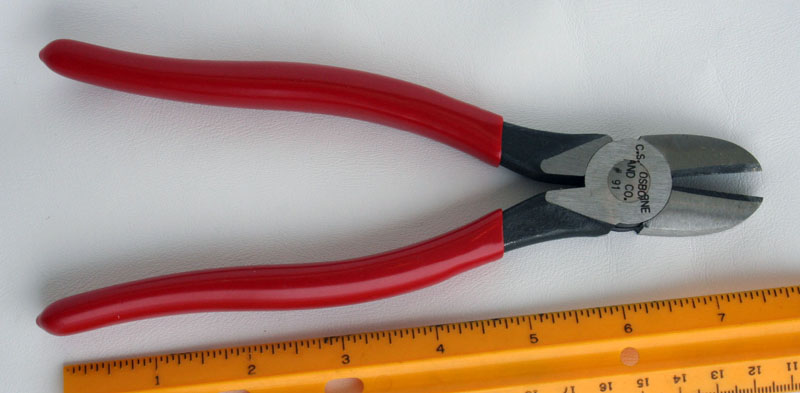The image depicts a pair of wire cutters, which are also referred to as snips. They feature red rubber-coated handles that transition to black towards the cutting part, which has a shiny metallic finish. There is a round metal piece just before the blade, inscribed with "C.S. Osborne" and "ANCO number 91," likely indicating the brand or manufacturer. The wire cutters are positioned next to a yellow ruler, used to measure their length, which is approximately 7.5 inches. The entire setup rests on a completely white background, possibly a sheet of paper or a white table, enhancing the visibility of the items for scale and detail.